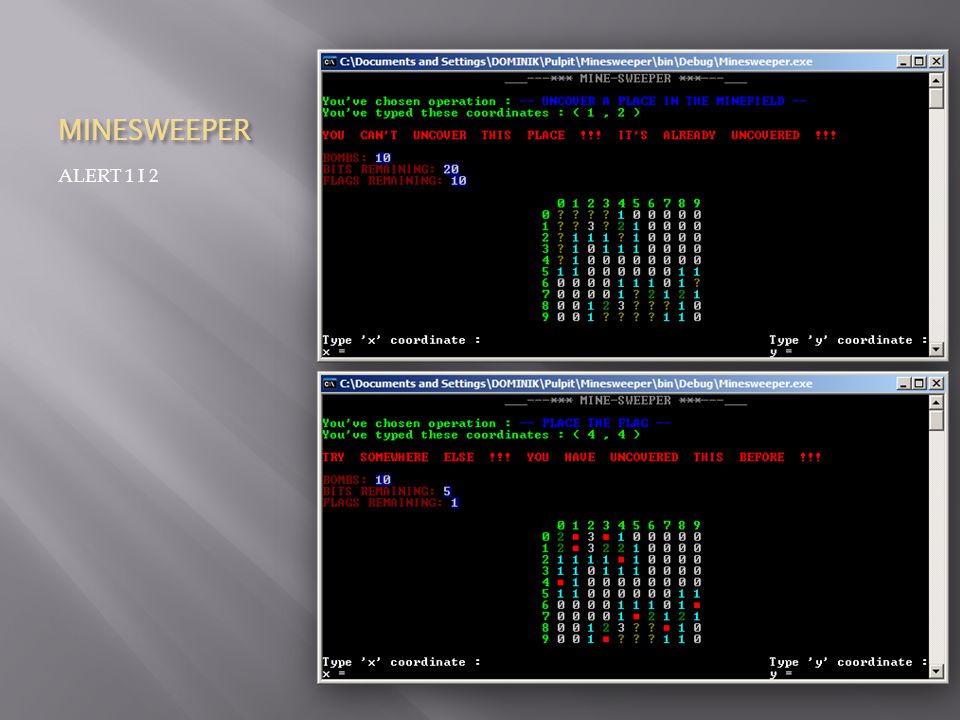The image shows two instances of the Minesweeper game running on a computer, encapsulated within a gray background that has a diagonal shading effect filtering from the left-hand side. Both Minesweeper windows, which possess an old MS-DOS and Windows 95 aesthetic, feature a blue upper border naming the program as Minesweeper.exe. The left-hand side of the image prominently displays "MINESWEEPER" in all-cap yellow font and "Alert 1T2" in white font just below.

The top part of the screen shows a detailed pathway, likely from a command line or file directory, displaying C:\drive\documents and settings\Dominic\pulpit\Minesweeper\bin\debug\Minesweeper.exe. Both Minesweeper games differ in their displayed states but share a mix of green, white, and light teal numbers indicating the proximity of mines, with text in green and red scattered across the interface. The text instructs players on various operations: "uncover a place in the minefield" and "place the flag," followed by specific coordinates like 1, 2 and 4, 4. Additional notes indicate what actions have been taken or are forbidden, such as "You can't uncover this place; it's already uncovered," and whether the coordinates have already been selected. One game display features red dots, while the other one does not. In the background, there's a black screen providing additional contrast to the Minesweeper windows and their colorful elements.